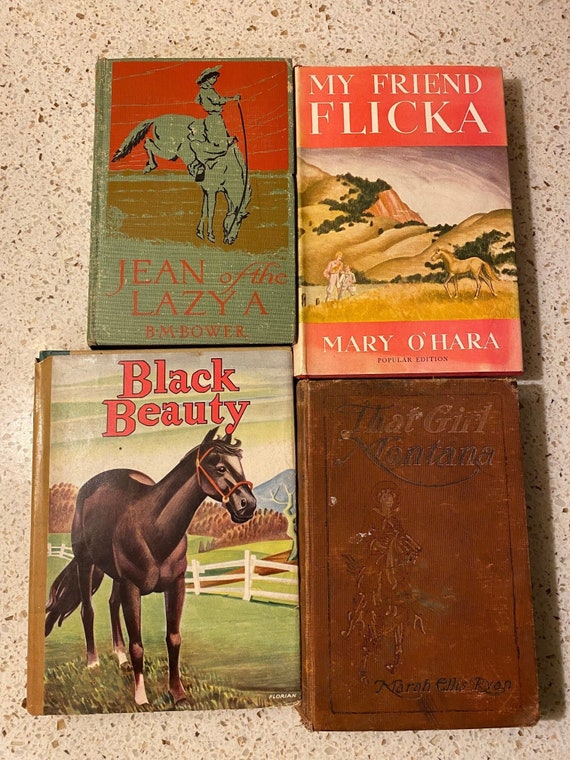The image features a set of four vintage hardcover books laid out on a weathered, buckled countertop, possibly made of textured stone or coral. These books appear to be quite old and show significant signs of wear.

The top-left book, "Gene of the Lazy A" by B.M. Bower, sports a green cover with red highlights at the top and the author’s name in red. The cover art depicts a woman in a western-style hat riding a horse that is bucking its hind legs, all set against a brown, dusty surface.

To the right of it, "My Friend Flicka" by Mary O'Hara, labeled as a popular edition, features artwork of rolling hills with a bay-colored horse walking in a field towards two people, likely a pioneer woman and a child.

On the bottom left lies "Black Beauty" with the name "Florian" in the bottom right corner of the cover. This book showcases a black horse with white markings on three of its hooves, standing on a green field with a white picket fence, distant hills, and a small tree in the background.

Completing the set, the bottom-right book, "That Girl Montana" by Mara Ellis Ryan, appears to be the oldest and is in extremely rough condition. The dark brown cover is scuffed and worn, barely revealing a faded illustration of a girl riding a horse, with the text almost illegible.

Each book likely portrays stories centered around horses, with a notable focus on female riders, reflecting a rich, equestrian heritage.